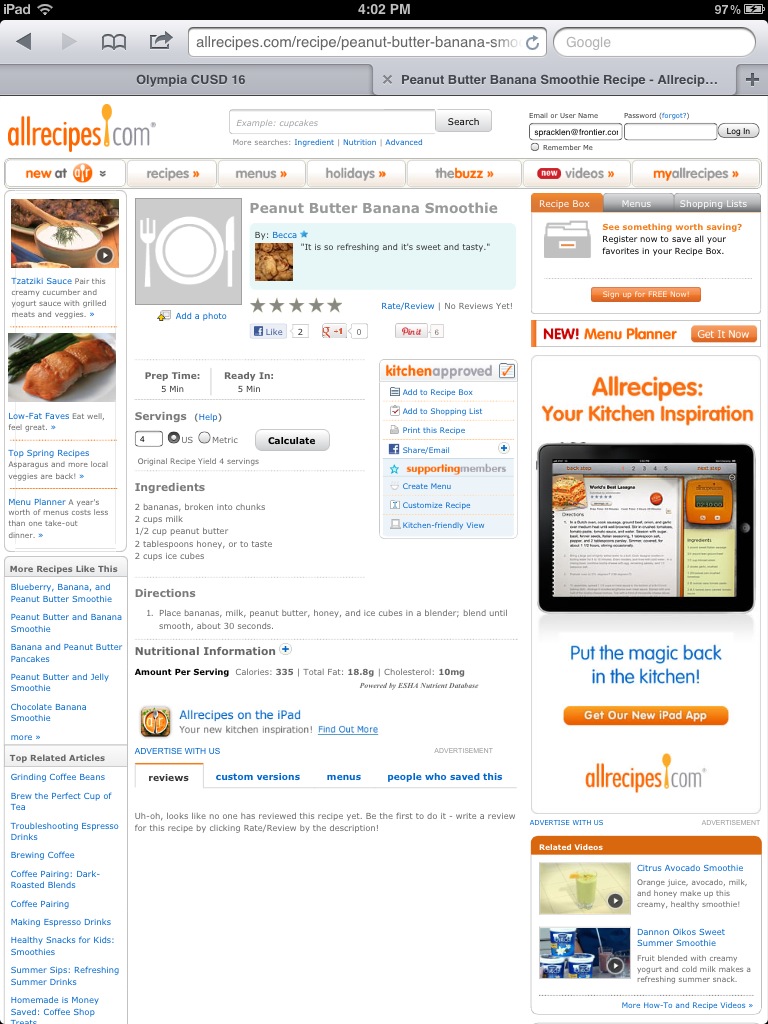This is a detailed color screenshot of the AllRecipes.com website displaying a recipe for "Peanut Butter Banana Smoothie." The screenshot is taken on an iPad, held in portrait orientation. At the very top of the screenshot, a black horizontal bar displays "iPad" in white text on the left, the time "4:02 PM" in the center, and a battery icon showing "97%" on the right. Directly below this, a gray browser bar features the URL "allrecipes.com/peanut-butter-banana-smoothie," with visible tabs including "Olympic CUSD 16" on the left and "Peanut Butter Banana Smoothie Recipe, All Recipes" on the right, which is the active tab.

The website's header includes the AllRecipes.com logo on the top left, where the dot in ".com" is depicted as a spoon icon, and the site name appears in orange text. A search box is positioned to the right of the logo, followed by various navigational tabs. 

In the center of the screen is the highlighted recipe, titled "Peanut Butter Banana Smoothie," which boasts a five-star rating. The ingredients listed include 2 bananas broken into chunks, 2 cups of milk, 1/2 cup of peanut butter, 2 tablespoons of honey or to taste, and 2 cups of ice cubes. The preparation instructions detail placing the bananas, milk, peanut butter, honey, and ice cubes into a blender and blending until smooth, roughly for 30 seconds. Nutrition information is also provided—each serving contains approximately 335 calories, 18.8 grams of total fat, and 10 milligrams of cholesterol.

Advertisements line the right column while additional links and content populate the left side of the page, completing the layout of this informative and visually appealing screenshot.